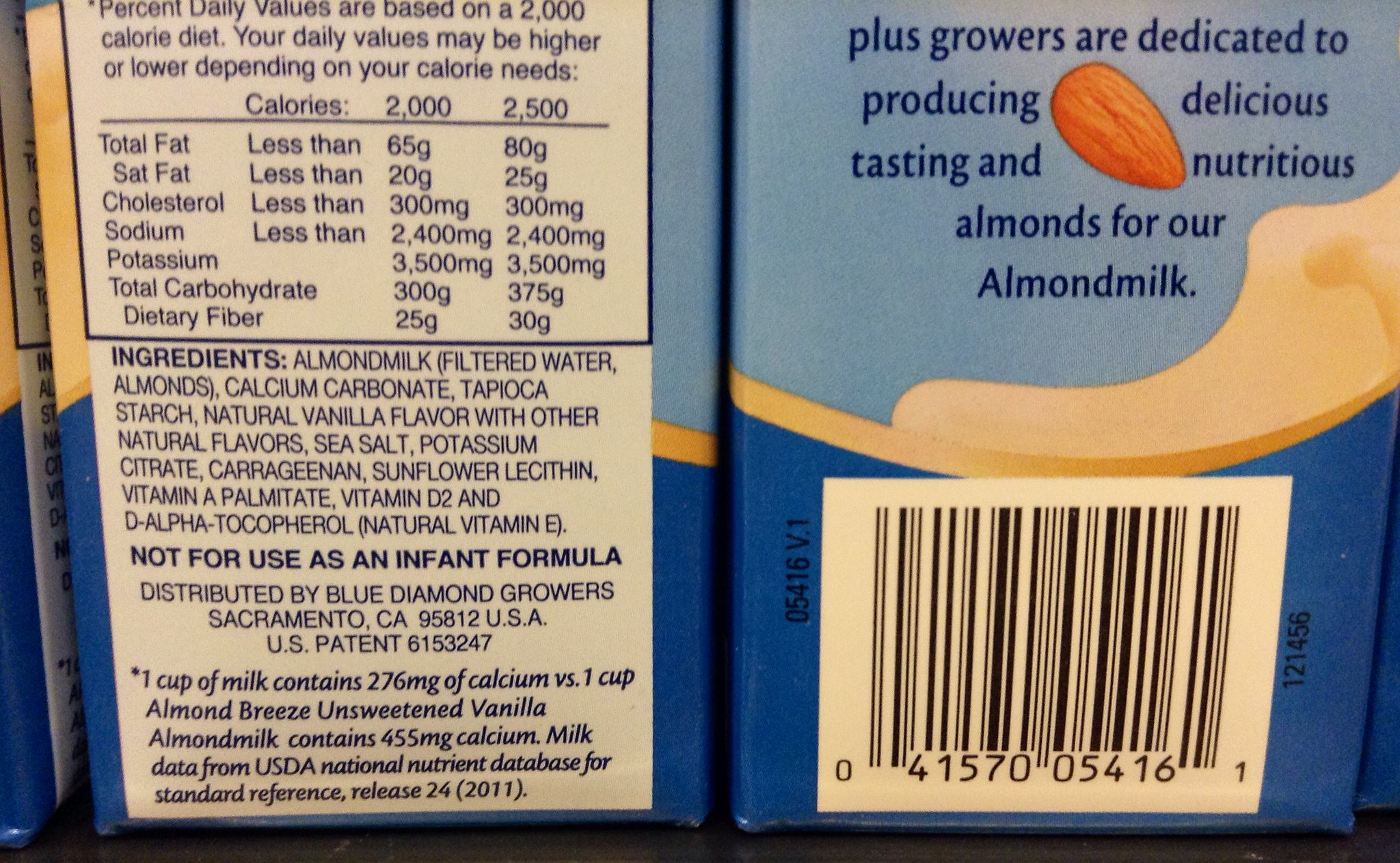This close-up photograph captures the sides of an almond milk carton, prominently showcasing its nutritional information and ingredient details. The carton is visually striking with a color palette that transitions from dark blue at the bottom to light blue towards the top, accented with gold. A picture of an almond with flowing milk adorns the middle, emphasizing the product's primary ingredient. 

On one side of the carton, a quote in elegant blue font highlights the dedication of the growers: "Our growers are dedicated to producing delicious tasting and nutritious almonds for our almond milk." Below this, there is a barcode with the number 41570054161.

The adjacent side of the carton lists detailed Nutrition Facts against a white background, specifying the daily values based on a 2000-calorie diet, including total fat, saturated fat, cholesterol, sodium, potassium, total carbohydrates, and dietary fiber. The ingredients are also listed in blue text: almond milk (filtered water, almonds), calcium carbonate, tapioca starch, natural vanilla flavor with other natural flavors, sea salt, potassium citrate, carrageenan, sunflower lecithin, vitamin A palmitate, vitamin D2, and D-alpha-tocopherol (natural vitamin E). A bold statement indicates the product is not for use as an infant formula. 

Further down, the carton provides the distributor's information: Blue Diamond Growers, Sacramento, CA 95812, USA. It also compares the calcium content of the almond milk to regular milk, supporting its nutritional claims with data from the USDA National Nutrient Database.